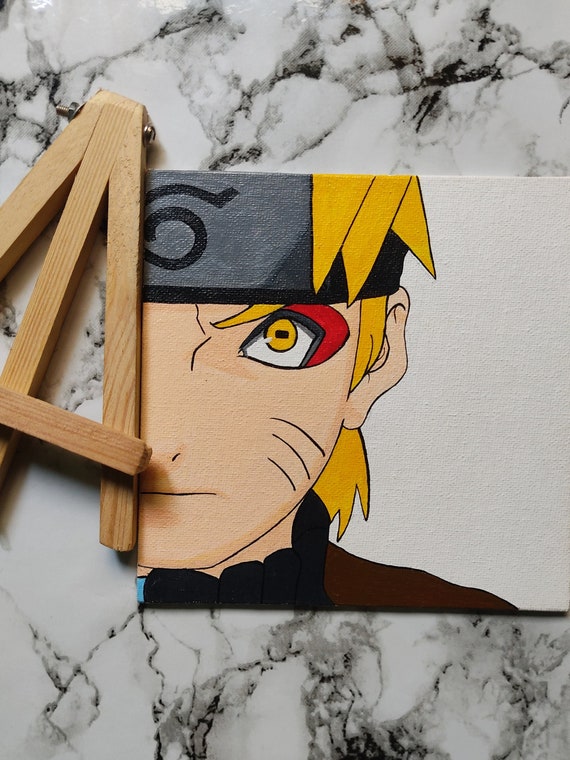A photograph reveals a small, square canvas painting of Naruto from the Japanese anime series, resting on a white and gray marble surface. The marble features intricate black veins adding texture to the mostly white stone. To the left of the painting is a partially visible, triangular section of what appears to be a wooden easel. This easel is used to support the small artwork. The painting itself captures only half of Naruto's face, focusing on one eye, part of the nose, half the mouth, and an ear partly concealed by yellow shocks of hair protruding from under a gray hat. A brown garment is visible just above his shoulder, along with black and a hint of turquoise blue around the neck area. The background of the painting is white, adding contrast to Naruto's vivid features and his concentrated expression. The canvas appears to be about the size of two credit cards, suggesting the painting may either be intentionally cropped or simply designed to display only this portion of the character.